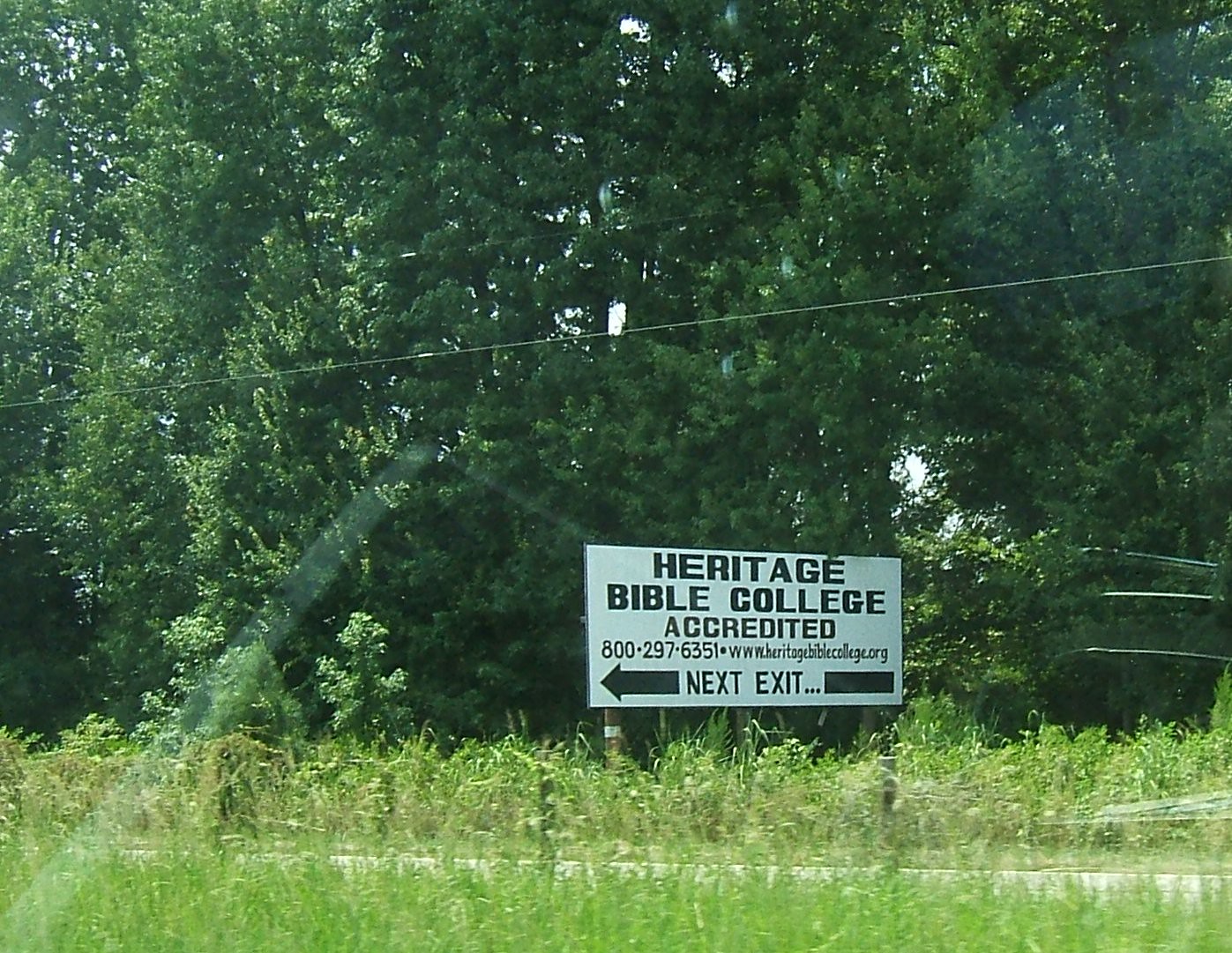The image captures an outdoor scene with a rectangular white billboard set against a backdrop of evergreen trees. The billboard has bold black lettering, prominently displaying "Heritage Bible College Accredited" at the top. Below this, contact details are provided: "800-297-6351" and "www.heritagebiblecollege.org." An eye-catching, thick boxy black arrow points to the left with the words "Next Exit" inside the arrow. The area surrounding the sign is lush with greenery, featuring tall grass in the foreground and a mixture of grass and possibly a path or street in front of the billboard. The evergreen trees behind the sign enhance the natural setting.